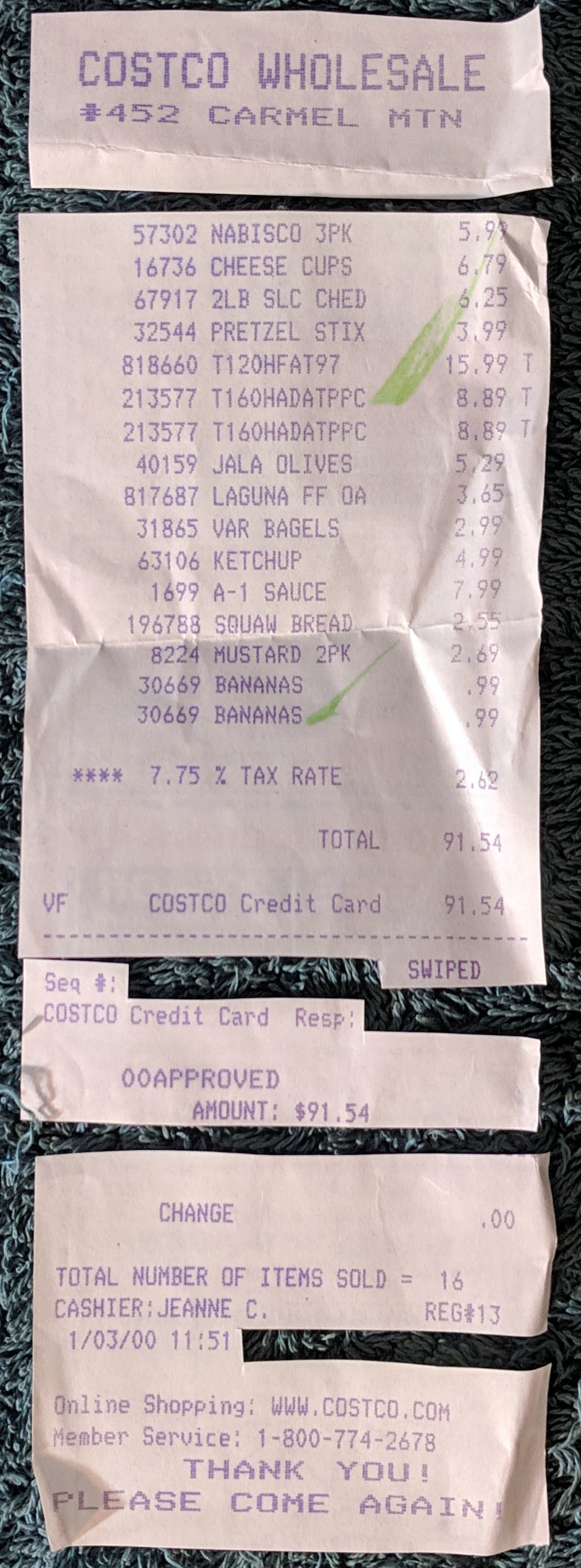This is a detailed photograph featuring a receipt from Costco, displayed against a table with a distinctive black and robin's egg blue pattern. The receipt, associated with Costco Wholesale No. 452 in Carmel Mountain, has been meticulously cut into four jagged pieces, possibly to remove personal information. The top segment identifies the store details: "Costco Wholesale No. 452 Carmel Mountain." The subsequent portion lists the purchased items, including two bunches of bananas, ketchup, and A1 sauce, along with a tax of $2.62. The total amount spent is $91.54, paid using a swiped Costco credit card, as indicated on the receipt. The cut segments display essential transaction details such as the sequence number, approved amount ($91.54), total number of items sold (16), and a message at the bottom reading "Thank you, please come again." Notably, there is a small rectangular piece missing from the middle of the receipt.